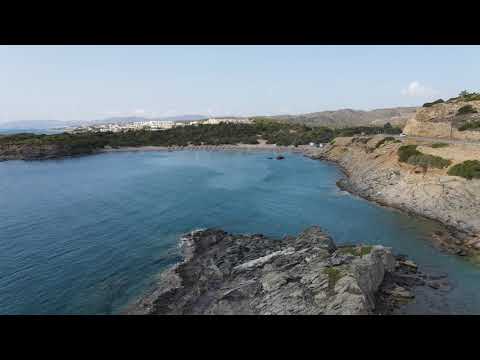This photograph, taken from an aerial perspective, showcases a dark blue lake dominated in the foreground by a massive, jagged rock formation resembling an island. The rock itself exhibits a rugged mix of white, gray, and black hues with patches of green seaweed or grass. Surrounding the lake are cliffs of gray, light brown, and tan rock interspersed with grassy patches. A road curves along the cliffs' edge where a car is visible, leading towards more rocky hills and mountainous terrain in the distance. Across the lake's edge, a rocky beach is present, bordered by large, lush green trees. Behind these trees lies a small city featuring white commercial buildings or warehouses. Further in the background, the scene transitions into more expansive brown and jagged mountains, topped by a light blue sky with a few clouds emerging from behind the distant peaks.